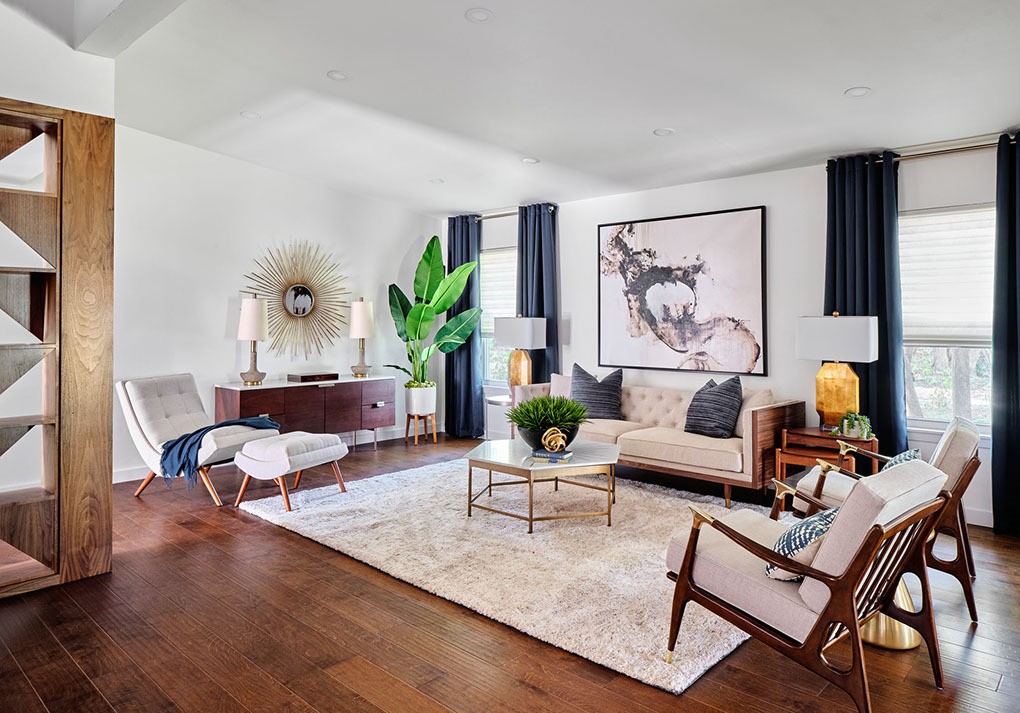The image depicts a modern living room with white walls and ceiling, featuring recessed lighting. The central focus is a beige cushioned sofa with wooden legs and sides, adorned with two blue pillows. Flanking it are two wooden end tables, each with a lamp. Above the sofa hangs a large painting. In front of the sofa, there is a six-sided table, possibly metal with a marble top, placed atop a beige area rug.

On the right side, two wooden chairs with cream-colored cushions are positioned beside a large window with open blue curtains. Adjacent to the chairs is a triangular end table with a lamp.

On the left side of the living room, there's a white lounge chair with an ottoman in front of a long console table. Mounted on the left wall is a mirror with a decorative gold sunburst pattern between two lamps, and a large green plant stands nearby.

The room has mid-century modern elements, with wooden furnishings and white or off-white upholstery, and a cohesive color scheme of blue, beige, and white.